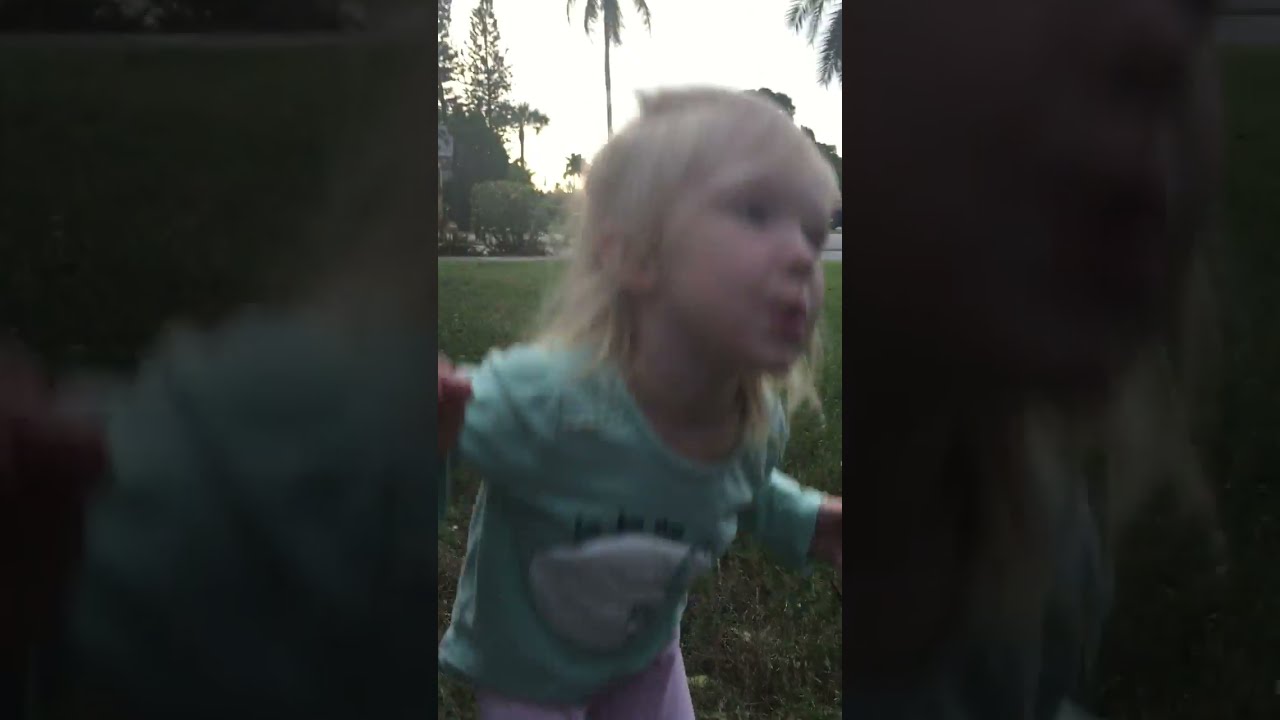The image centers on a young girl, possibly around three years old, who is looking towards the right. She has blonde, shoulder-length, straight hair and appears to be making a puckered-up kiss face. She is wearing a light green, long-sleeved t-shirt with a white graphic, potentially depicting a sheep, and purple (or pink) pants. Her hands are clenched into fists in front of her. The background features a green lawn with short grass, various bushes with green leaves, and tall trees, including palm trees in the top right and top left corners. The sky is light gray, indicating daytime. The photo composition includes the center image clearly, while the left and right thirds are darkened and blurred versions of the center.